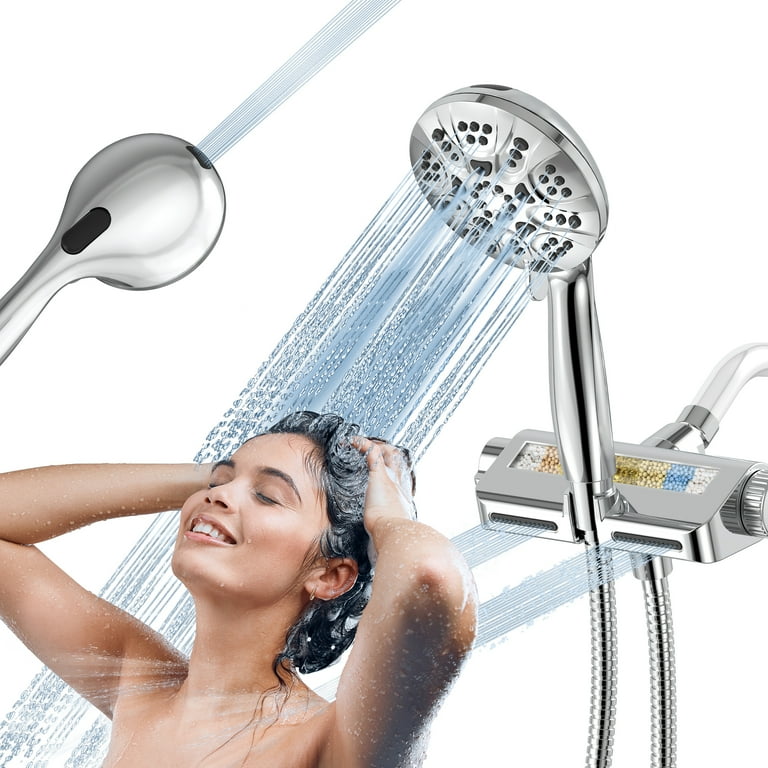A sleek advertisement showcases a versatile shower system featuring multiple sophisticated showerheads. At the center, a large, round handheld showerhead is mounted in its holder, cascading a soothing stream of water onto a woman. This oversized showerhead offers a luxurious bathing experience. Surrounding the main showerhead, several additional water jets emit evenly spaced streams of water, enhancing the overall coverage.

Innovatively integrated into the showerhead holder, various bath beads can be seen, suggesting an infusion of aromatherapy for a spa-like experience. In another image, a silver showerhead features an alternate mode that acts like a high-pressure hose, capable of delivering several concentrated jets of water for a more vigorous rinse. Overall, this dynamic shower system is designed to provide a customizable and refreshing shower experience, blending relaxation with functionality.